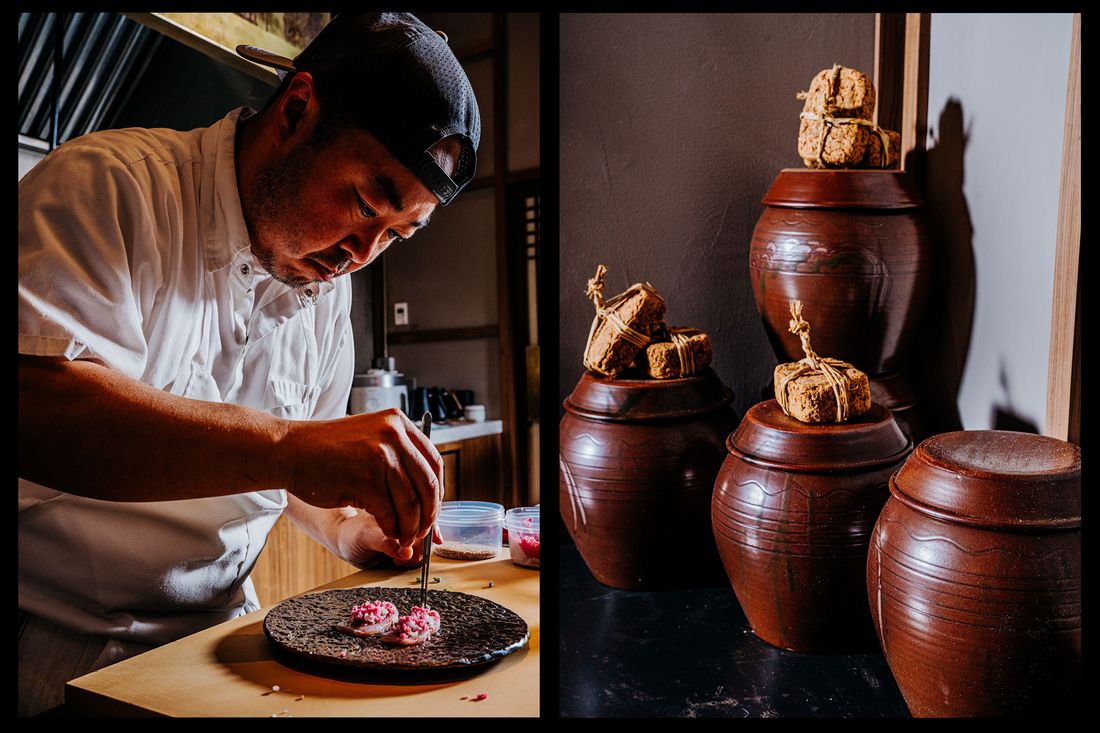The image depicts an Asian chef, with a mustache and serious expression, meticulously putting the final touches on a culinary dish. He is wearing a backwards black baseball cap, a white chef's shirt, and an apron. Using tweezers, he is carefully placing small red garnishes onto two round, pinkish items that resemble either sushi or deviled eggs. These items rest on a craggy, textured stoneware plate situated on a kitchen counter. In the background, there are two containers holding different ingredients, one of which contains the red garnishes. To the right, the scene transitions into an adjacent image showing five large brown ceramic jars with simple designs and ceramic lids. Three of these jars have ropes tied around large stones or bricks placed on top, possibly for fermenting purposes like making kimchi.